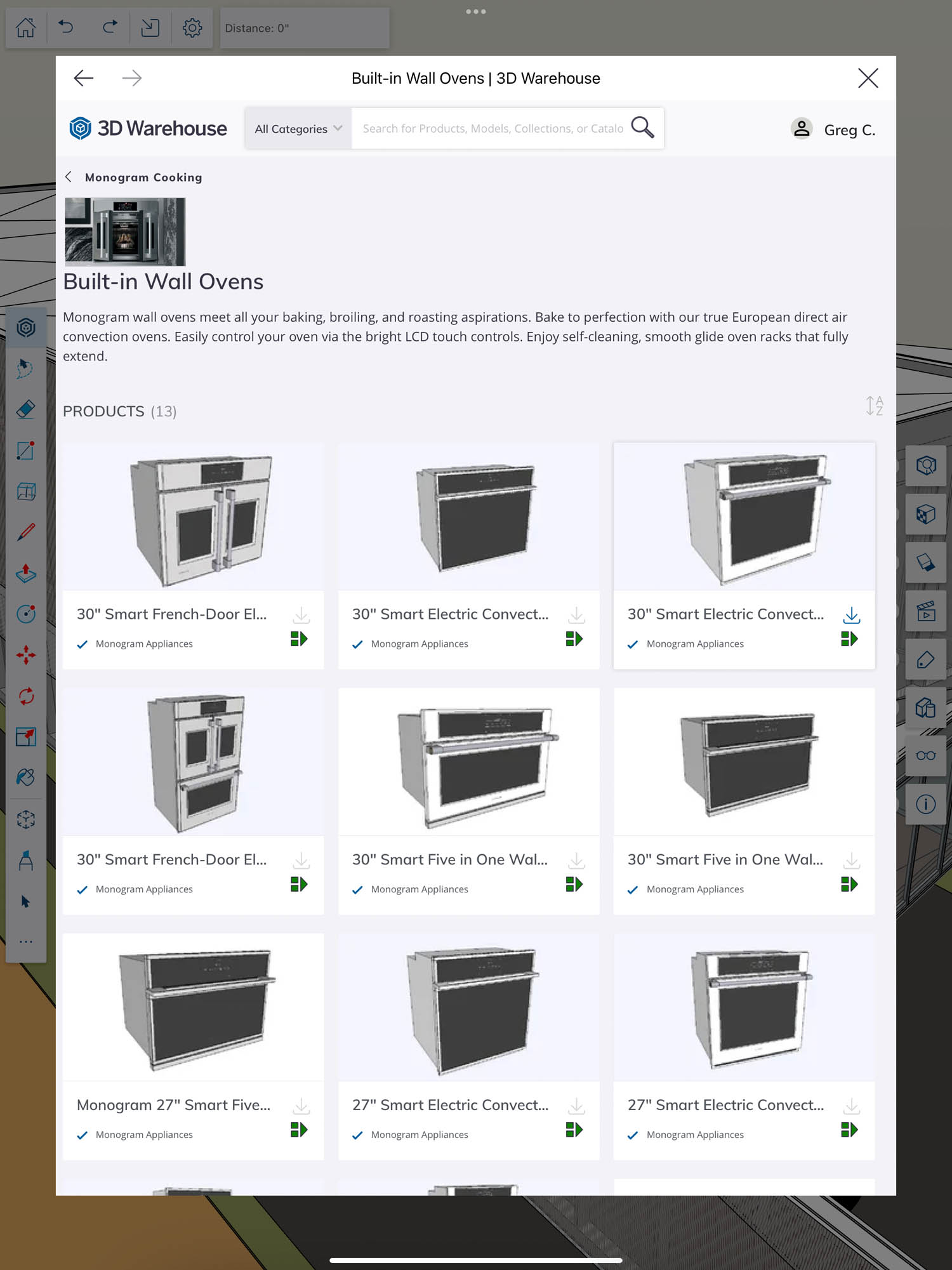This is a screenshot of a web page with a secondary pop-out window in focus. The background page displays various icons at the top left, including a home icon, a left arrow, a right arrow, and a text box that reads "Distance: 0". To the left side of the screen, there's a vertical toolbar featuring icons such as an eraser, a pencil, a marker, and an arrow. On the right side, another list of icons includes twelve square boxes and a clapboard, typically used in film production.

At the center of the image, the pop-out window prominently features the text "Built-in Wall Ovens 3D Warehouse" in black. There's a logo alongside the title "3D Warehouse," a search bar labeled "All Categories," and the username "Greg C." Below this header, there's a section displaying "Built-in Wall Ovens" with a small preview image and a brief paragraph of information. Additionally, three rows showcasing three different oven models each are featured, with corresponding images and titles beneath each oven.